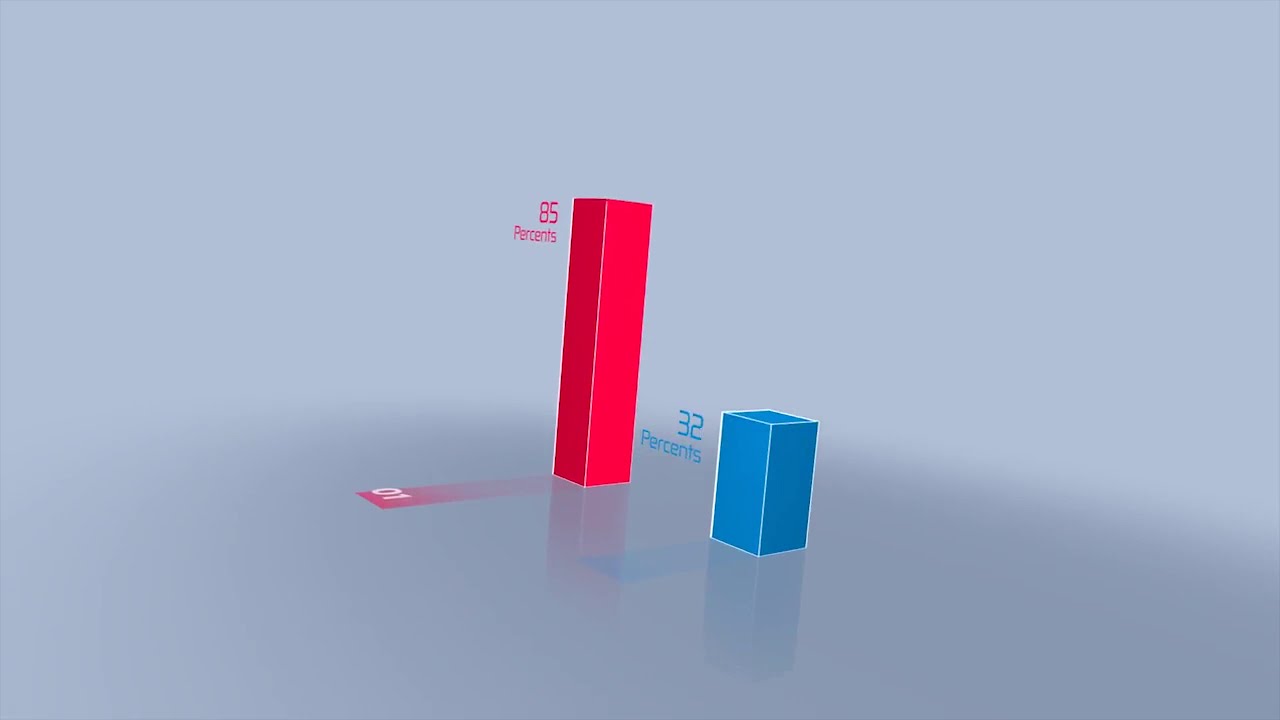The image features a digital, three-dimensional bar graph set against a gradient gray background, transitioning from light gray at the top to dark gray at the bottom. The graph consists of two central vertical bars: a taller, vibrant red bar on the left labeled 85%, and a shorter, bright blue bar on the right labeled 32%. Both bars cast corresponding colored shadows in front of them—red for the red bar and blue for the blue bar. While the shadow of the red bar also shows a slight, faint red reflection containing the number "10," no reflections are reported for the blue bar. There are no additional elements, text, or information within the image, making the focus solely on the contrasting percentages and colors of the bars against the gray backdrop.